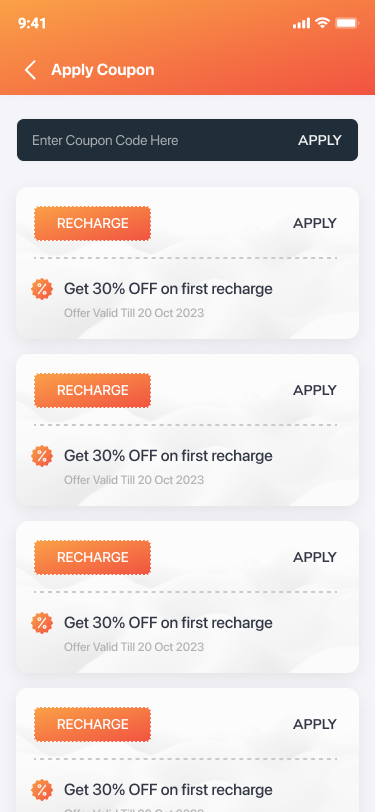The image is a screenshot taken from a mobile phone displaying an application designed for purchasing and applying coupons online. The app appears to be focused on offering discounts for a product or service that requires periodic recharges, indicating that the user incurs a cost with each recharge. The interface primarily features an orange and white color scheme, giving it a clean and modern look. At the bottom of the screen, there is a search bar where users can enter and apply a coupon code. Below the search bar, there are multiple selections of coupons, with four visible in this screenshot. Each coupon includes a "recharge" button accompanied by an "apply" link to the right. Additionally, there is text underneath stating, "Get 30% off on first recharge," affirming the benefit each coupon offers. While the screenshot reveals various details about the functionality and design of the app, the name of the app is not visible in the image.